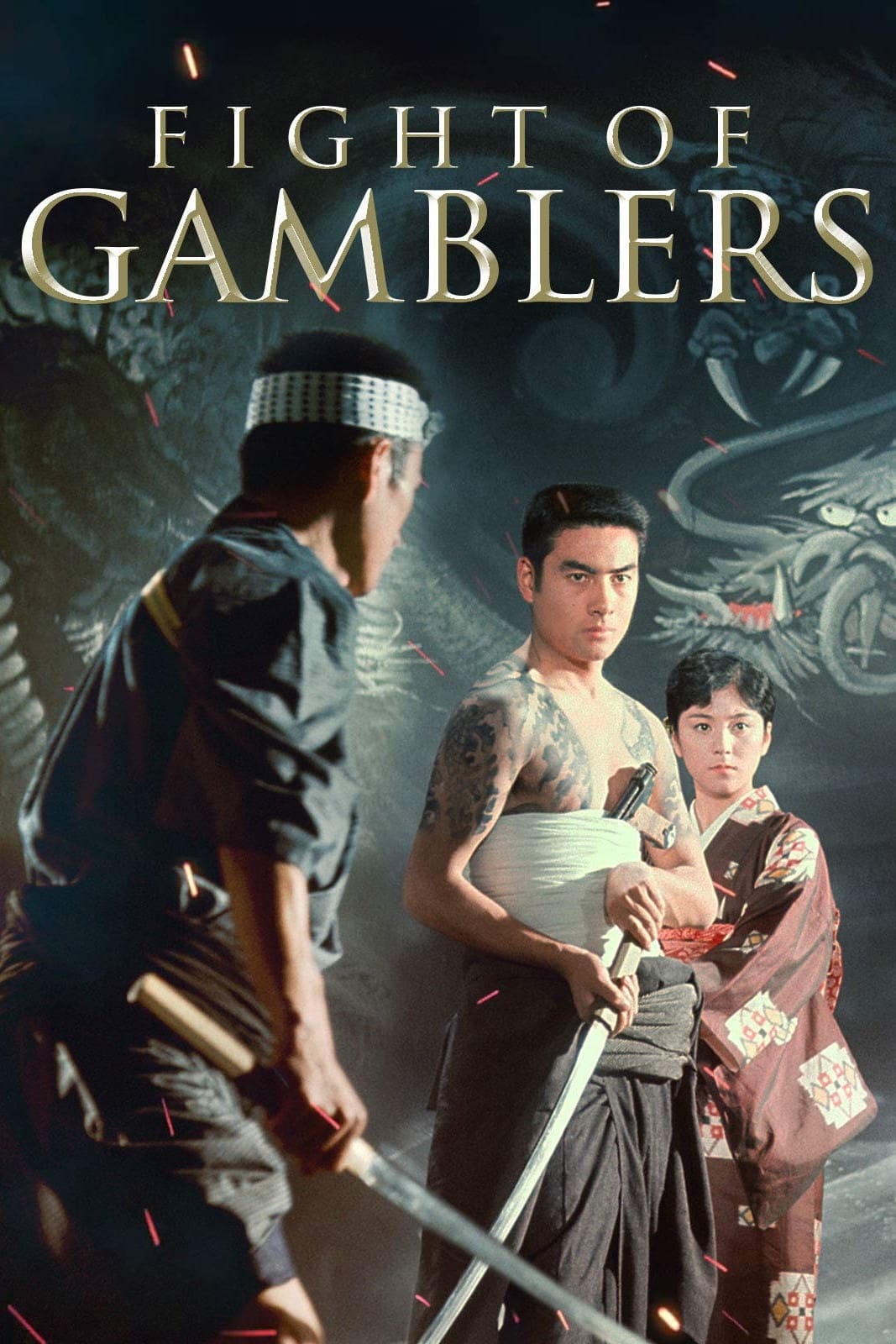The image, a dynamic blend of color illustration and graphic design with photographic elements, presents a dramatic indoor scene titled "FIGHT OF GAMBLERS," displayed prominently at the top in bold, metallic lettering. Set against a dark backdrop adorned with Chinese dragons, the central focus is on two Japanese warriors poised for combat, each holding samurai swords pointed downward. 

On the left stands a Japanese man, his intense gaze directed almost toward the camera. He is shirtless, revealing a canvas of intricate tattoos across his shoulders and torso. His midsection is wrapped in a white sash, securing a weapon—possibly a gun or sword. He wears dark grey baggy pants, exuding an aura of raw strength and provocation. 

Opposite him, facing slightly away from the viewer, is another man wearing a traditional tunic in shades of white, black, and grey. His attire includes a headband of matching colors, and he appears composed, gripping his sword with readiness. 

Behind the tattooed warrior, a Japanese woman stands in a dark red and white kimono, with intricate gold motifs. She looks concerned, her eyes directed to the right side of the frame. The complex backdrop, featuring meticulously designed dragons in shades of grey, adds a mythic and intense atmosphere to the scene. Scattered throughout the image are small, striking red dashed lines, enhancing the overall graphic composition.